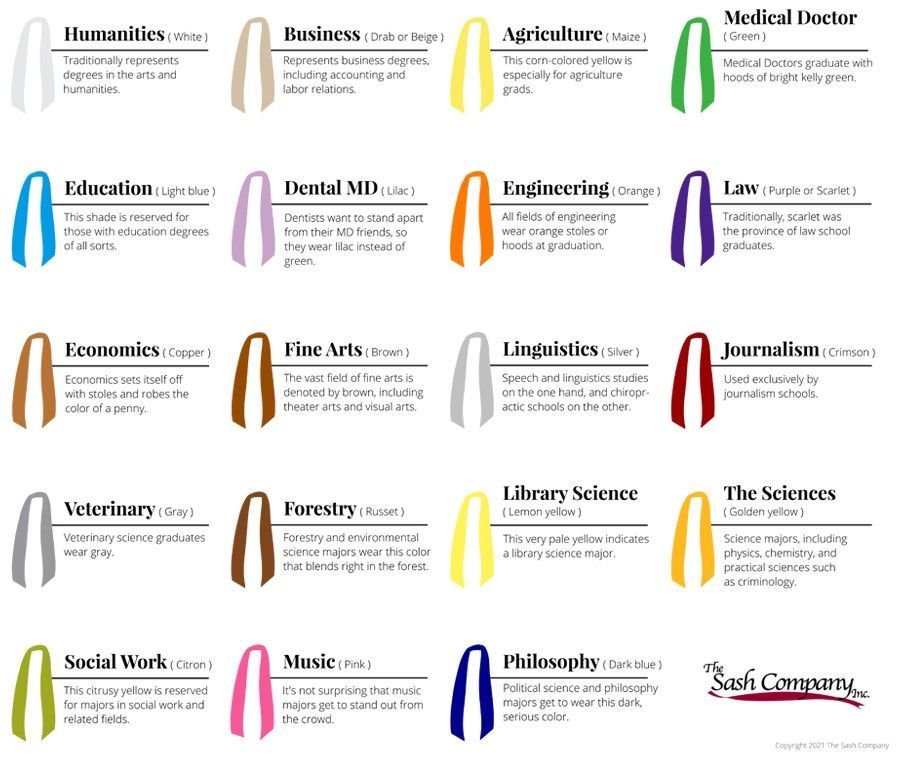The image is an infographic displaying an array of sashes used for college graduation, with each sash representing a different major through distinctive colors. Arranged from left to right and top to bottom, the majors and their corresponding sash colors are as follows: Humanities (white), Business (brown), Agriculture (yellow), Medical Doctor (dark green), Education (blue), Dental MD (pink), Engineering (orange), Law (purple), Economics (copper), Fine Arts (dark brown), Linguistics (red), Journalism (crimson), Veterinary (gray), Forestry (russet), Library Science (lemon), The Sciences (golden yellow), Social Work (citron), Music (pink), and Philosophy (light blue). These sashes are displayed against a clean white background. On the bottom right corner of the image is the logo and name of the company, "The Sash Company Incorporated". Directly beneath the logo is a dark red or maroon-colored sash.